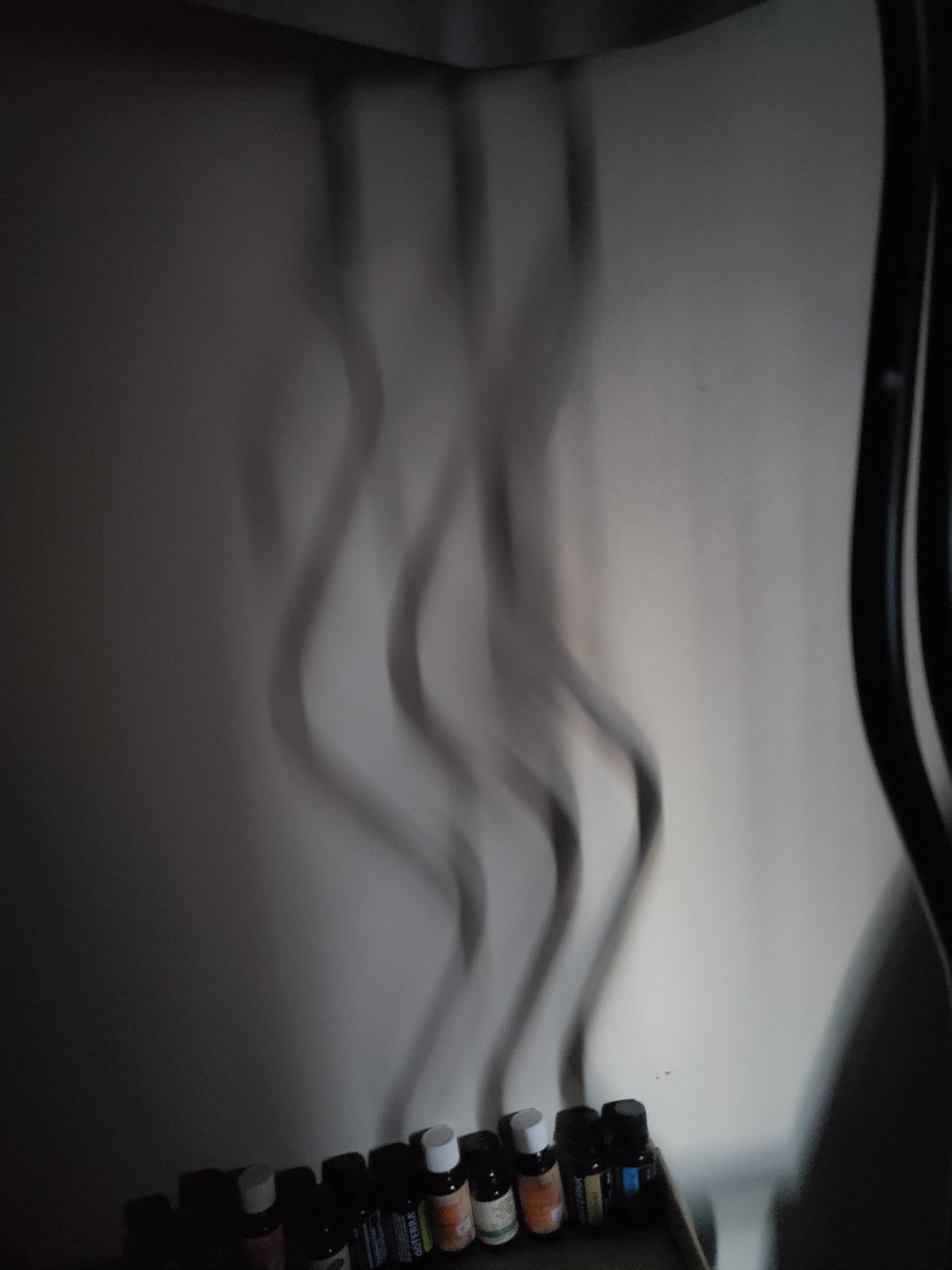Amidst a soft, dreamlike blur, the image centers around an intriguing arrangement of cables or wires casting dramatic shadows. These shadows trace a graceful, serpentine path from the top, curving down to the left, then swinging to the right, and finally converging in the middle. Below this shadowed interplay, a collection of glass bottles fills the scene. Their caps vary in color: black, white, and others, contributing to a mosaic of orange, green, yellow, and black labels that hint at an assortment of contents. The backdrop is a pristine white wall, which subtly enhances the contrast. On the right side, a section of wavy wood adds texture and depth, shrouded in shadows. The entire image is wrapped in a soft focus, rendering its elements into an almost abstract portrayal, leaving the viewer's imagination to fill in the details.